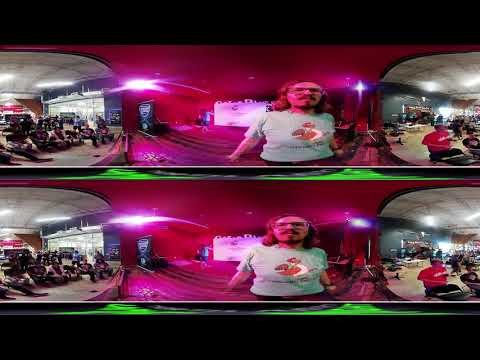This is a double image, one stacked on top of the other, each featuring the same blurred, reddish-pink lit room with a neon glow. The central subject across both images is a Caucasian man with long, light-colored hair reaching his shoulders. He wears glasses, sports a full mustache and goatee, and dons a blue t-shirt with a cartoon chicken graphic—white chest, tan feathers, and a brown tail. The top image shows the man turned slightly to his left in a three-quarter angle, while the bottom image captures him from the front. On either side of the man and the reddish room are oval or circular areas with a gray backdrop, which resemble an airport terminal or waiting room. These areas are populated with people and appear cluttered, with spaces featuring gray ceilings and floors. The overall composition creates a rounded, warped effect, reminiscent of a photograph taken with a panoramic or fisheye lens.